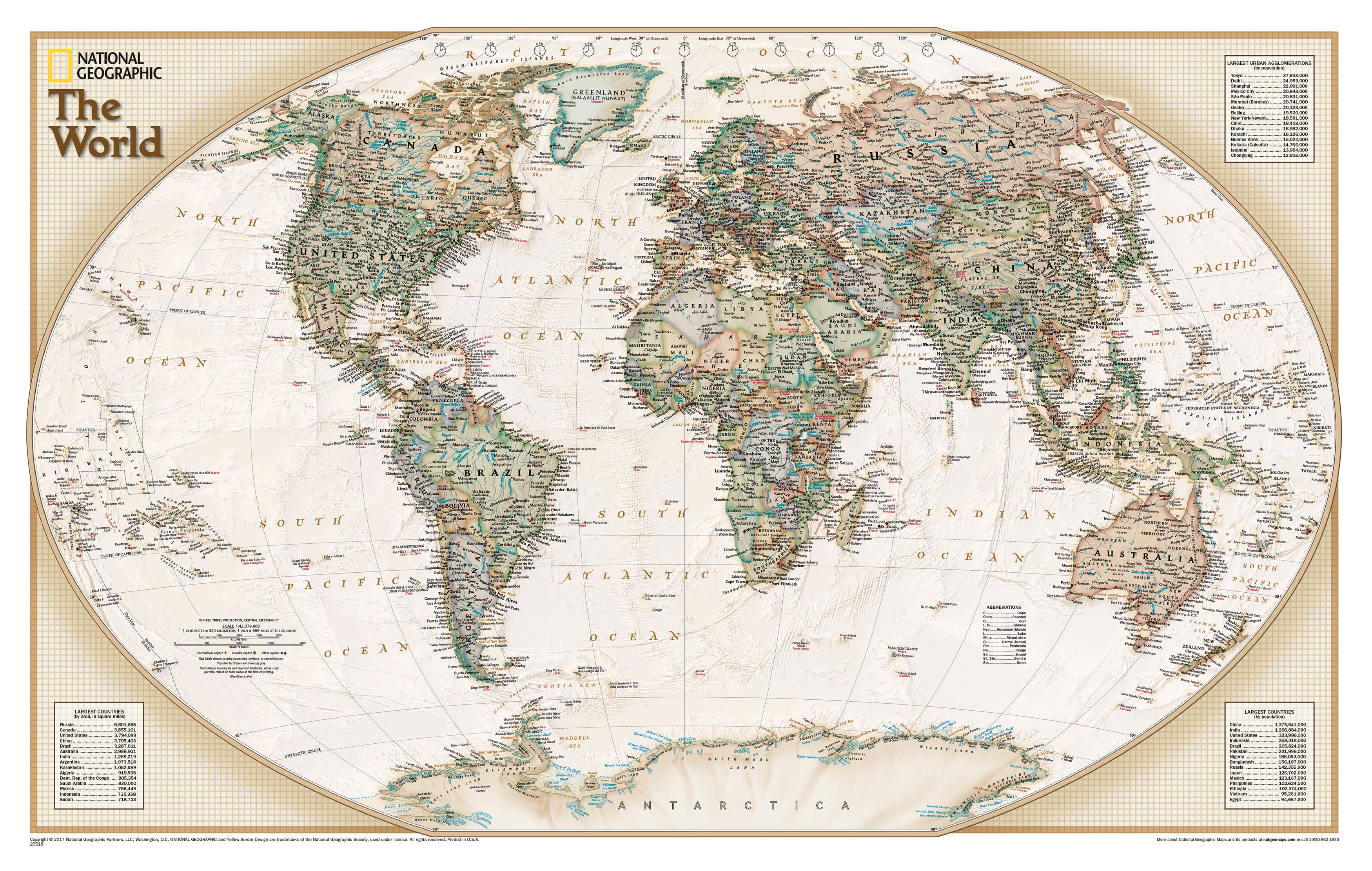This rectangular image showcases a world map created by National Geographic, prominently labeled in the upper left-hand corner with "National Geographic" and "The World" just below. The map features a detailed, flattened depiction of the globe, highlighting all continents and major bodies of water. North America, South America, Africa, Europe, Asia, and Australia are all clearly visible, with Antarctica stretched across the bottom of the map and Greenland near the top. The continents are depicted in various colors to outline different countries and borders, though the font of the country names is small and difficult to read. The names of oceans, including the North Pacific Ocean, North Atlantic Ocean, and Indian Ocean, are clear. The image also includes a legend or key in the bottom left, bottom right, and upper right corners, although the small font makes these labels hard to decipher. The map itself is predominantly in beige and white tones, providing contrast for the detailed geographic features and making the text and outlines stand out against the background.